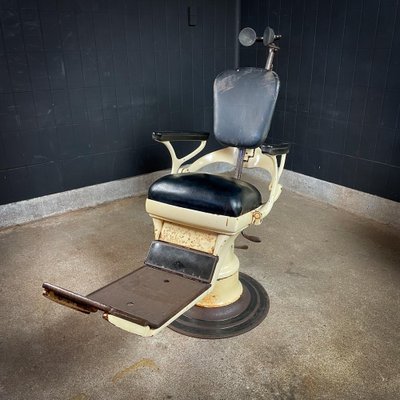The photograph captures an old-fashioned dental chair in an empty indoor room with visible signs of wear. The room features dark blue, scuffed walls with white trim at the bottom, and a concrete floor that may have once been carpeted. The chair itself is primarily blue with black seat cushions and armrests made of thick black leather or vinyl. The chair's metal components are an off-white or ivory color, showing some rust, and include a substantial circular base that suggests it might be fixed to the floor rather than mobile. At the front of the chair, a large footrest made of grayish-black metal extends outward, and there are pedals at the back for adjusting its height. The setting and the equipment suggest a vintage dental practice, highlighted by the distinctive headrest composed of a metal bar and circular supports on either side.